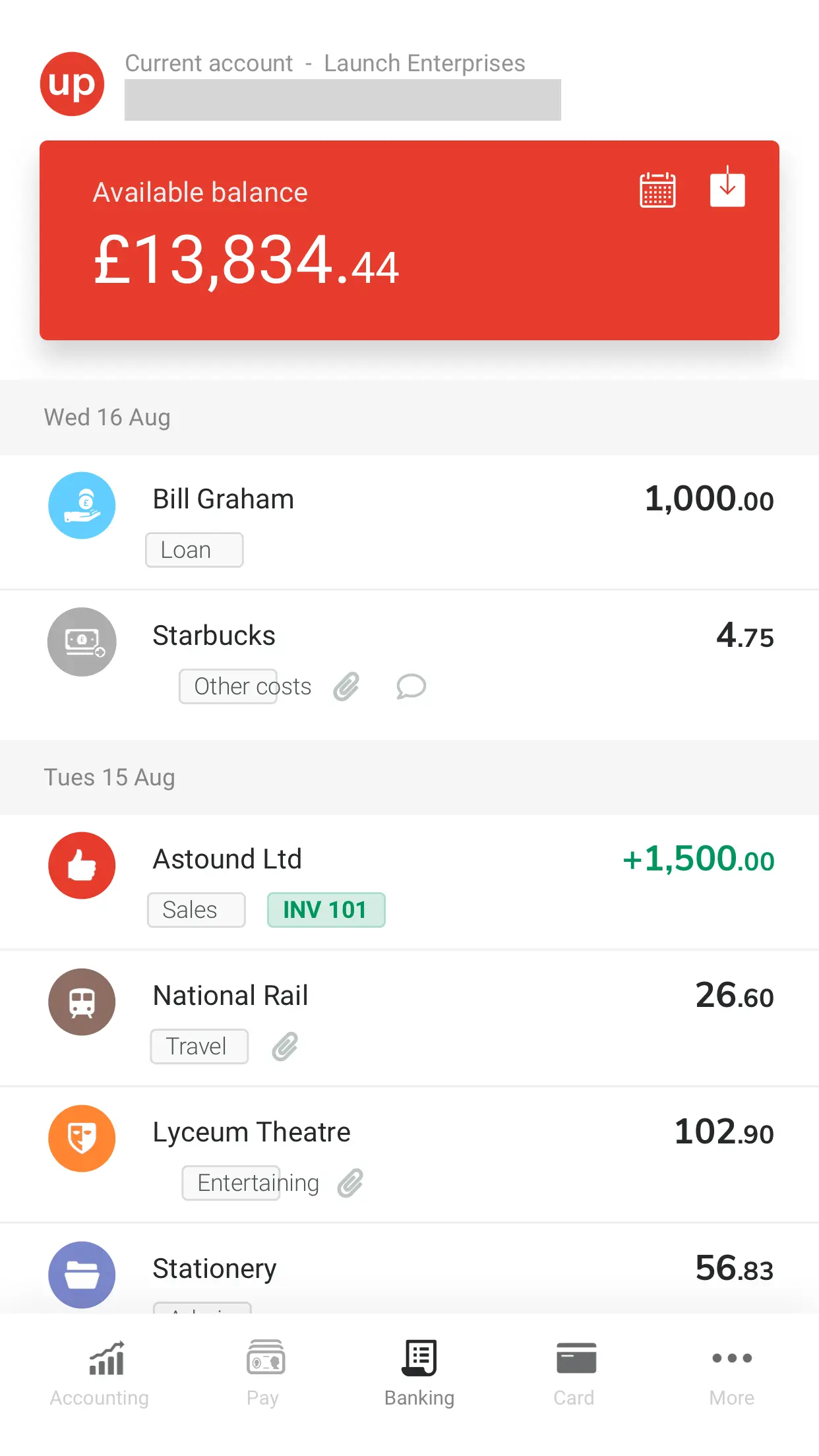The image appears to be a screenshot from a smartphone displaying a financial account summary. At the top left corner, there is an orange circle with the letters "UP" in white, adjacent to which is a gray bar. Above this, the text "Current Account Launch Enterprises" is visible. Below this header, there is an orange rectangular bar spanning the width of the screen, which displays the "Available Balance: £13,834.44," indicating the amount in British Pounds.

Underneath the orange bar, a gray border displays the date "Wednesday, 16 August." Below the date, two financial transactions are listed. The first transaction is for an individual named Bill Graham, indicated by a blue circle to the left. Adjacent to Bill Graham's name is a section labeled "Loan," specifying an amount of $1,000. The second transaction is labeled "Starbucks" under "Other Costs," showing a charge of $4.75 to the right.

A gray band beneath these transactions marks the date "Tuesday, 15 August," and four transactions are detailed below. The first transaction is from "Astound LTD," showing an addition of £1,500. The second entry is from "National Rail," with a charge of £2,660, categorized under travel expenses. The third item is for "Lyceum Theatre," amounting to £102.90, described as entertaining. The final transaction is listed as "Stationery," costing £456.83.